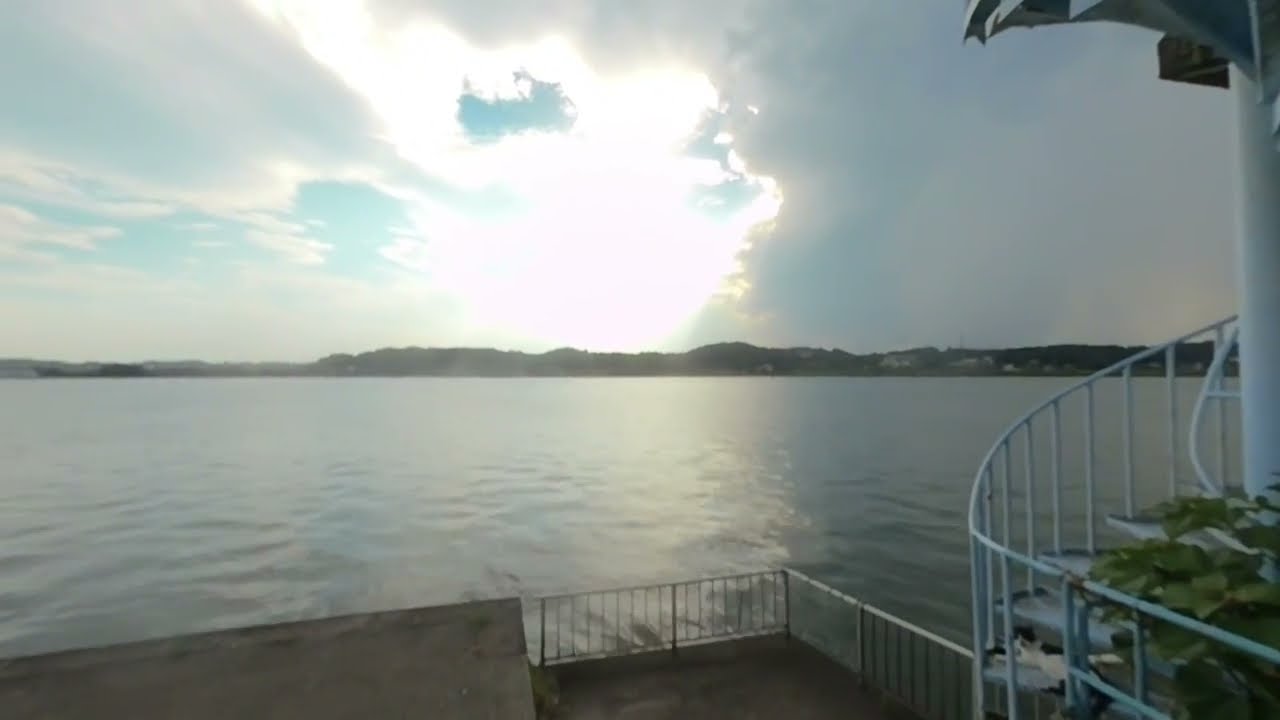The image captures a tranquil, expansive view of a large body of water—perhaps a lake, river, or ocean—taken from an outdoor location, possibly an apartment building or a restaurant. The scene is veiled in a gray, slightly out-of-focus haze, lending a soft, muted quality to the photograph.

The water stretches calmly across the bottom half of the frame, with faint ripples marring its stillness. On the distant horizon, a line of low, dark hills (possibly brown or black) can be seen, with some greenery and a few buildings scattering the landscape. Faintly, the outline of a boat appears on the far left side.

In the foreground, a deck with white fencing extends toward the water, juxtaposed with a metal hand railing forming a right angle near a concrete paved area. To the right, a spiral staircase, painted blue, winds upward around a white or light blue pole, leading to an archway that hints at a covered area. Plant leaves peek into the frame from the bottom right corner.

The sky is predominantly cloudy, with shades of dark gray accumulating on the right. A bright, white sun sits in the center of the sky, its rays piercing through the dense clouds, illuminating brief patches of blue. The light casts an ethereal glow over the entire scene, contributing to its overall serene and contemplative atmosphere.